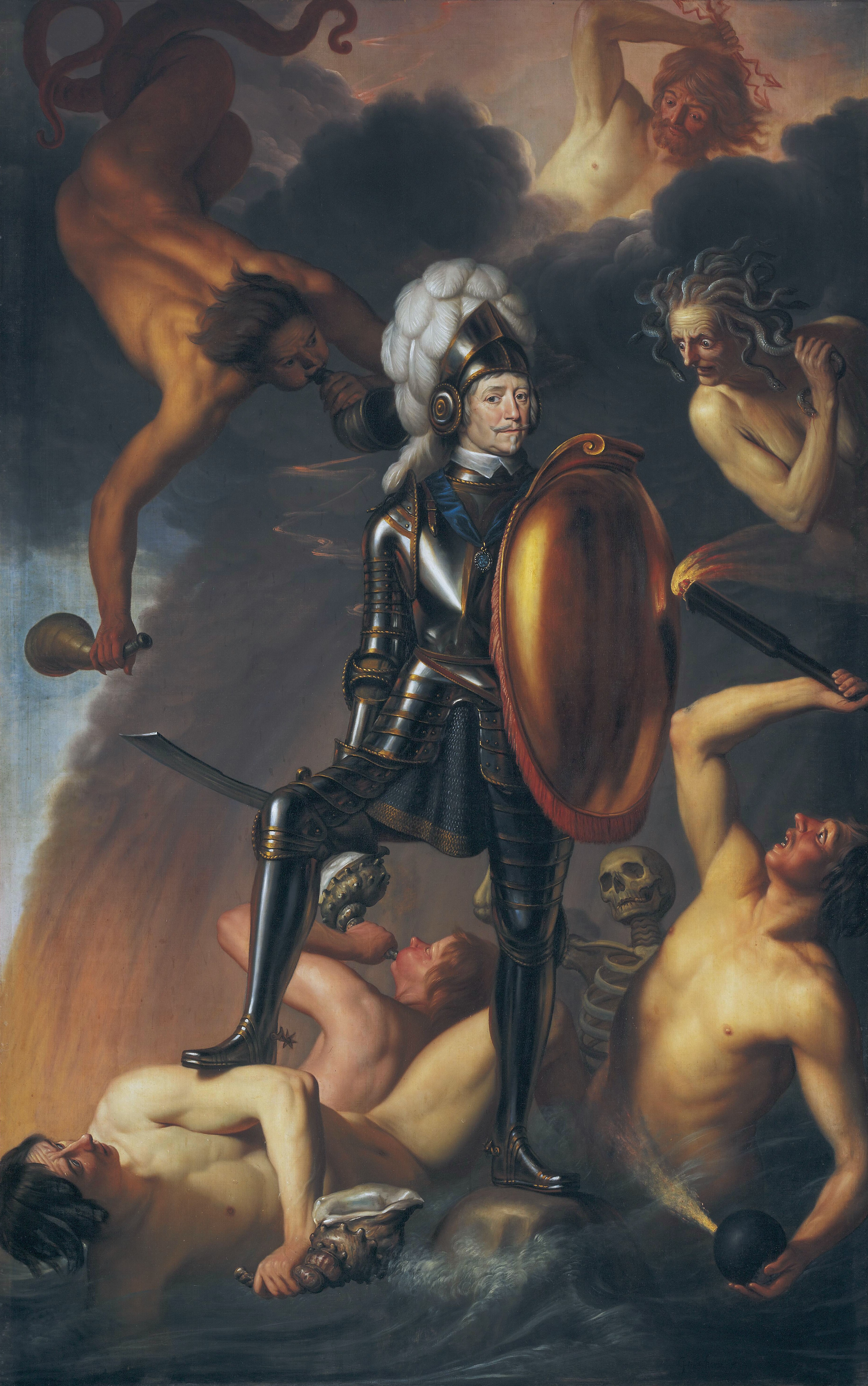The image depicts a rectangular oil painting featuring a central figure of a Caucasian knight or soldier in an elaborate, shiny bronze and blue suit of armor, adorned with a helmet that has white feathers behind it. The visor of the helmet is raised, revealing the man's face as he looks directly at the viewer. In his left hand, he firmly grips a large, oval, bronze-colored shield, while in his right hand, he holds a sword positioned behind his right knee. The soldier's right foot is assertively placed on top of a nude man who is holding a conch shell; this second man is partially submerged in a tumultuous gray sea, symbolizing defeat or subjugation.

Surrounding the armored soldier are a total of six additional figures, most of whom are mostly or entirely nude. In the waves below, there are two more men and a skeletal figure who appear to be emerging from or struggling within the sea. The skeletal figure is looking directly up at the soldier, adding a macabre element to the scene. To the left of the soldier, another figure holds an orb or bomb emitting sparks, poised to strike the soldier's shield, highlighting the chaotic and intense struggle.

In the sky above the scene, celestial or supernatural beings are depicted among dark gray and slightly orange clouds. On the left side, a figure is suspended by tentacle-like forms while blowing into a horn. To the right, a Medusa-like woman with snakes for hair gazes directly at the soldier, and nearby, another male figure, possibly Jesus or an angel, raises a thunderbolt as if ready to strike. These figures add a mythological and ethereal dimension to the painting, suggesting themes of divine intervention or cosmic justice.

The dark, stormy clouds and the roiling sea beneath enhance the overall atmosphere of conflict and epic struggle within the artwork.